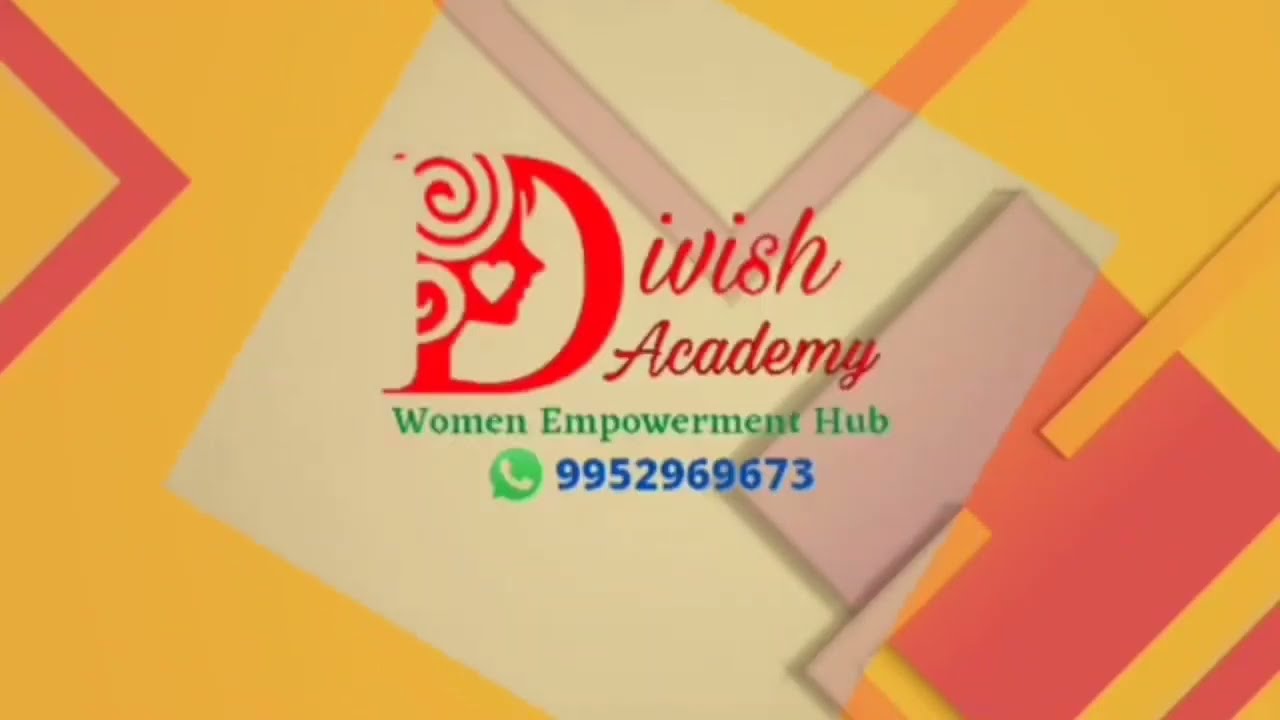The image is an advertisement for "Divish Academy" or "Dwish Academy," prominently featuring a large, ornate red letter "D," which is stylized with a woman's face, a heart on the cheek, and spiral designs forming the base of the letter. Below the "D," the text "Women Empowerment Hub" appears in green. The overall design includes a bold color scheme of yellow and red with overlapping geometric patterns like diamonds and rectangles. A semi-transparent, beige square overlay showcases the main text. The advertisement includes a green icon resembling a speech bubble with a phone in it, alongside the contact number "995-296-9673" in blue. The background integrates an interplay of light and dark orange, with intricate shapes creating a visually engaging display that implies empowerment and connectivity.